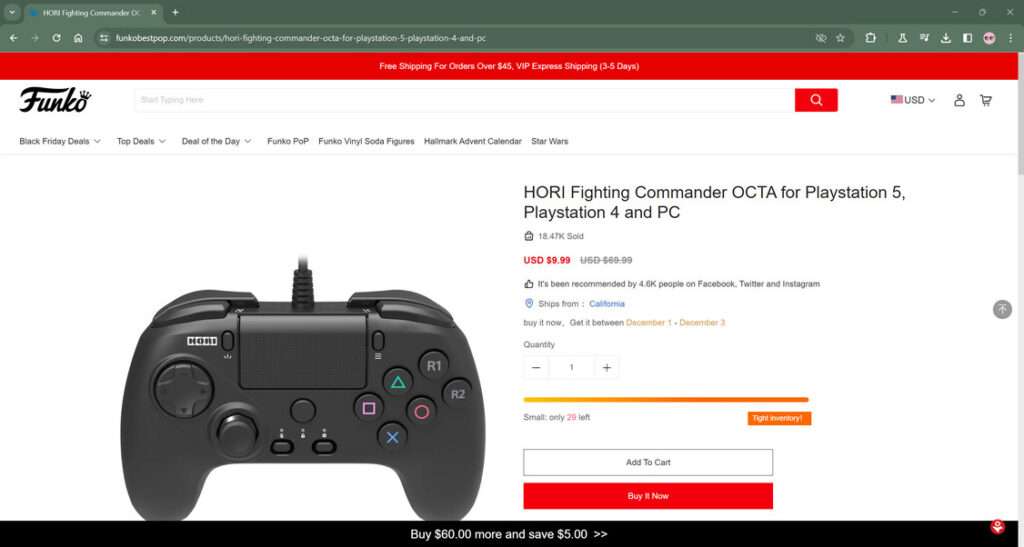**Website Navigation Interface**

At the top of the website, there is a grey bar featuring a search bar, although the text within it is not visible. This grey bar also contains navigation buttons including a back arrow, a forward arrow, a refresh button, and a home button. A star icon is available for bookmarking the page. Additionally, there is an option to download items. A pink smiley face wearing sunglasses is displayed as the profile picture. In the top right corner, there are three vertical dots indicating more options.

Below the grey bar, a prominent red banner announces "Free Shipping for orders over $45." Underneath this banner, the Funko logo is displayed, with a small crown adorning the letter "O." Another search bar is located below the Funko logo, displaying the text "USD" and accompanied by a small person icon and a shopping cart icon.

In the main content area, which has a white background, there is a large image of a black controller featuring various buttons: a blue X, a pink square, a pink circle, and a green triangle. The product is identified as "Hori Fighting Commander O.C.T.A for PlayStation 5, PlayStation 4, and PC" and is priced at USD $9.99.